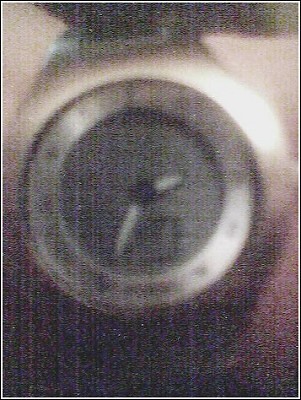This is a detailed and grainy close-up photograph of a wristwatch on a light-colored skin person's wrist, possibly taken from an old magazine due to its low resolution and grainy texture. The watch features a shiny metallic housing with silver and bronze or brass accents. The outer face is silver, encircling a darker gray inner face. The hour markers appear as dark, indistinct markings. The watch hands are white with black outlines, connected to a black central circle. One hand points towards the 2 and 3 o'clock position, while another extends towards the 7 o'clock position. The background, characterized by peach and red hues, suggests it is the skin of the wrist wearing the watch. The watch band seems to be made of linked silver components. Overall, the image quality makes finer details difficult to discern, but the watch's general form and features are identifiable.